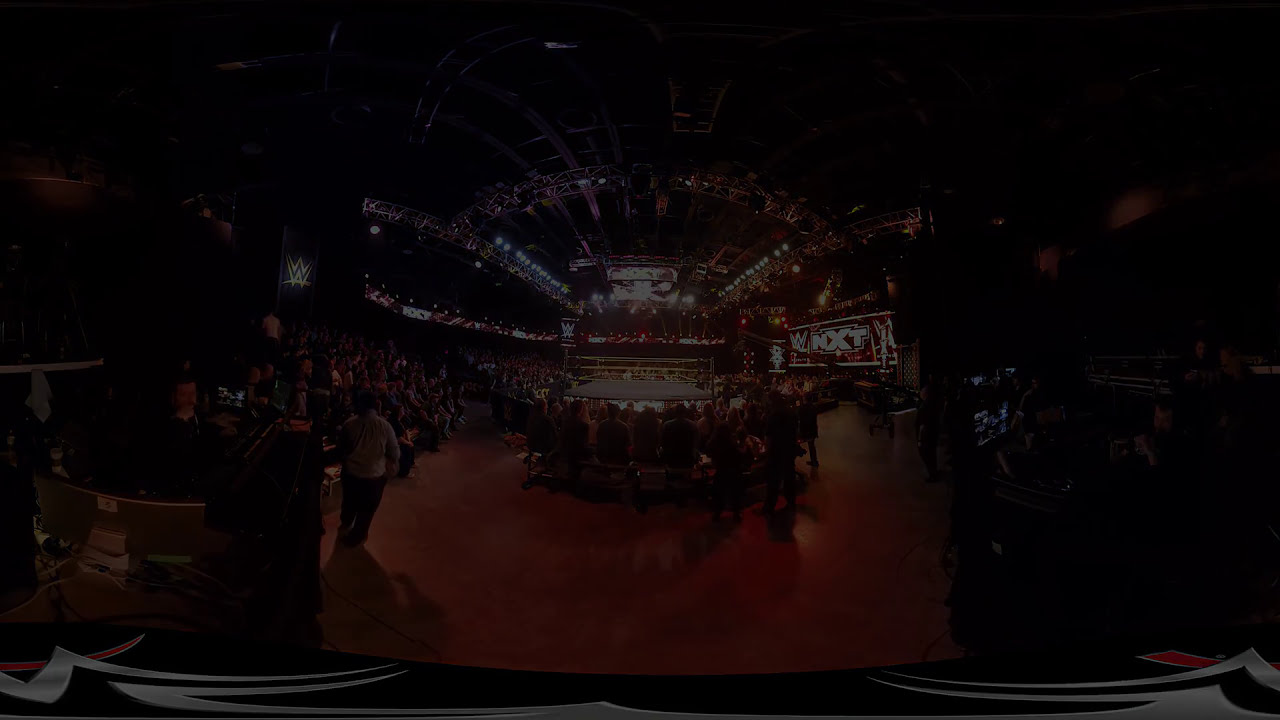The image captures a dimly lit venue, possibly an event such as a boxing match, UFC fight, or wrestling match inside a building. The focal point is a light-gray ring or stage in the center, surrounded by a crowd of spectators seated in the foreground and along both sides. The ground beneath the crowd is a dark orange and reflects faint light. Overhead, there are exposed steel rafters along with multiple rows of spotlights, casting a feeble glow onto the scene below. A set of white-lettered signage, one of which appears to read "NXT," flanks the ring on the left side. On the right, in the distant background, is a rectangle resembling a stained glass window with white and orange lights. The walkway is outlined by sharp white corners on a black and white carpet, creating a stark contrast to the overall darkness of the image.